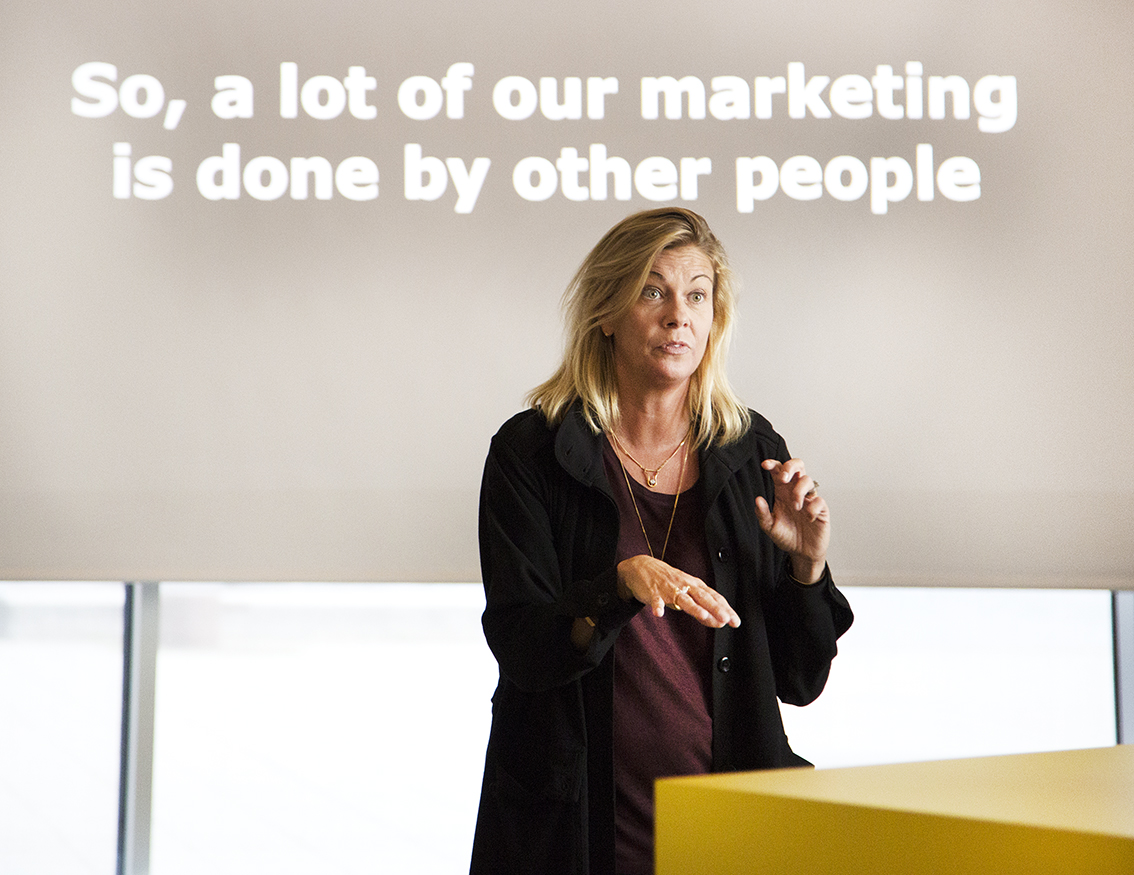A slightly older woman, possibly in her late 40s or early 50s, is giving a talk in what appears to be a business school or university setting. She has shoulder-length blonde hair brushed back, hazel eyes, and slightly parched lips with a hint of her teeth showing. Her face shows a surprised expression, emphasized by her raised thin eyebrows and noticeable wrinkles. She’s wearing a black jacket over a maroon or red blouse, and she has two gold necklaces; one with a pendant visible above her shirtline and the other hanging lower behind her hands. One of her hands is at chest level, and the other is extended outward, displaying a ring. The background features a light brown screen with white bold text that reads, “So a lot of our marketing is done by other people,” held up by two silver bars. A yellow box sits in the bottom right corner of the image, and a white wall with a shadow and a silver frame is visible on the left side.